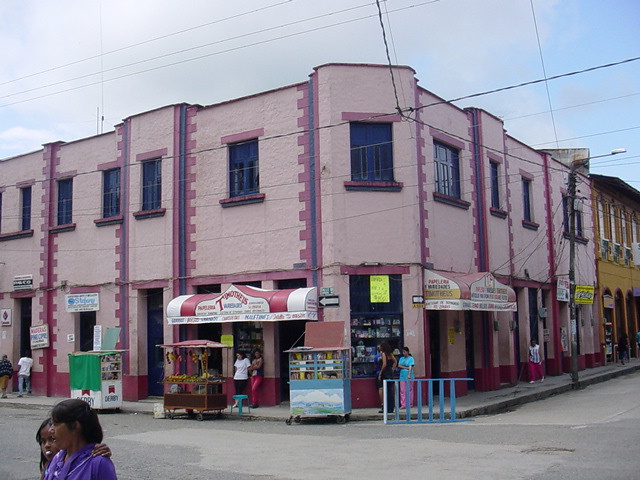This vibrant image captures a colorful two-story building situated on a street corner, extending downward along each side of the intersection. The structure is predominantly painted in shades of pink and purple, with a notable distinction between the lighter pink inner sections and darker pink, almost purplish, outer sections. The building's edges and trims are accented with even darker streaks of purple, emphasizing its unique and lively appearance. 

On closer inspection, the windows on the second story are framed with a bluish tint, while the first story features a series of storefronts adorned with awnings. Display cases in the corner storefront showcase various items, presumably including fruits and other goods, adding to the building’s bustling commercial vibe. Outside, a few carts, likely from the same store, are stationed at the front, suggesting active shopping and local commerce.

The scene is brought to life by the presence of several people milling around, either window shopping or walking along the sidewalk. In the lower left corner of the image, a woman in a purple shirt stands closely with a girl, possibly her daughter, adding a charming human element to the scene. Power lines crisscross the sky above, subtly indicating the setting's rustic urban feel.

The photograph also captures the transition from the pink and purple building to an adjoining yellow building on the far right, framed by a blue sky with a patch of white cloud. Below, the light gray pavement of the street appears patchy, further hinting at the character and age of the neighborhood.